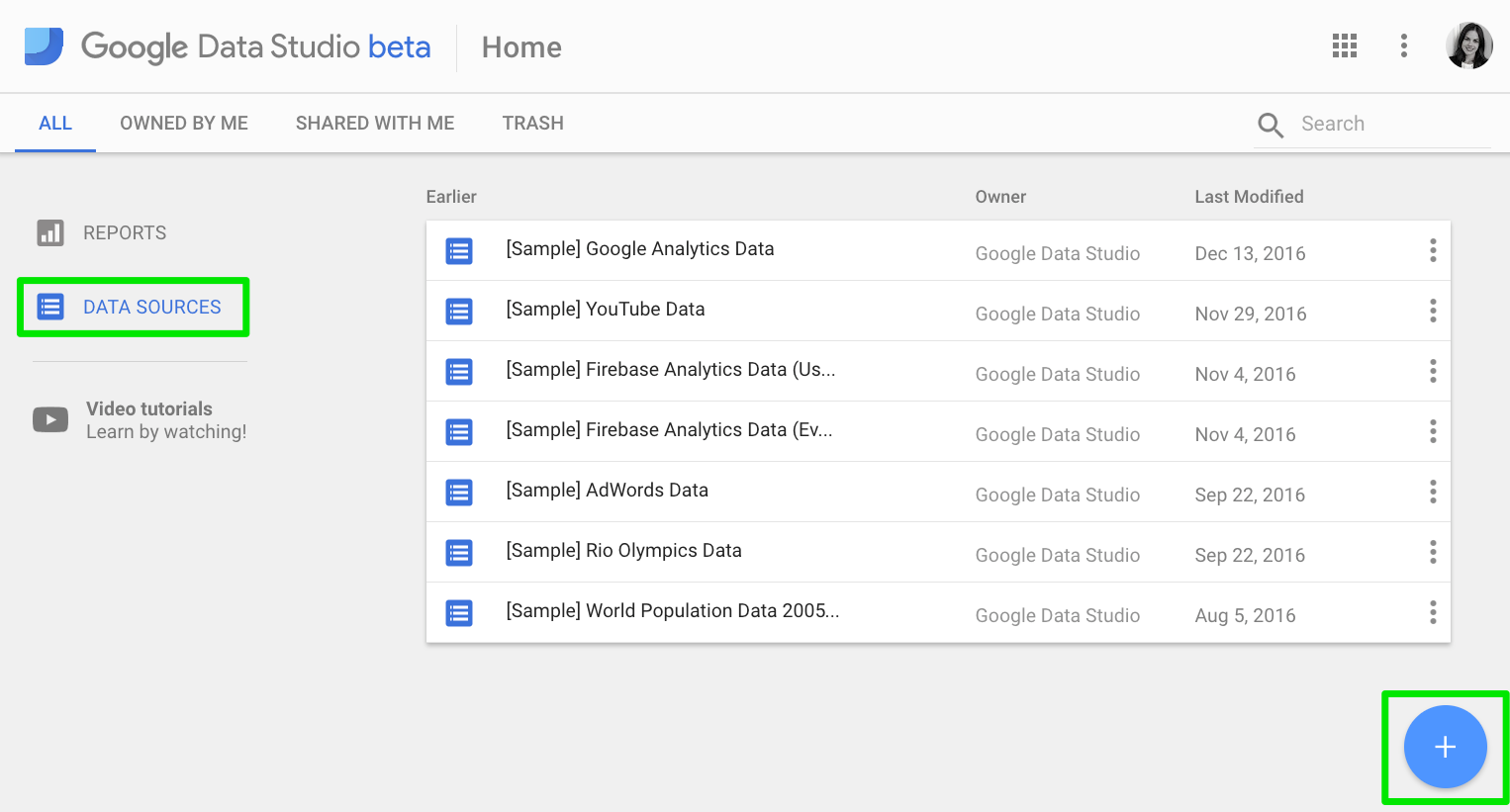At the top of the screen, there is a header that reads "Google Data Studio Beta" in a mix of black and blue text, accompanied by a light blue and dark blue Google icon. To the left of the header, it says "Home."

On the right side, there's a white bar with gray font. This bar includes several icons: squares, three dots, and a circle profile picture depicting a woman's face. Below this, there are navigation options in blue and gray: "All" in blue, "Owned by me," "Shared with me," "Trash," and a search bar with a magnifying glass icon next to it.

Continuing down the page, the menu lists:
- "Reports" in gray, accompanied by a small graph icon.
- "Data Sources" in blue, with an icon resembling a sheet of paper with white lines.
- "Video Tutorials" in gray, featuring a play button icon and the text "Learn by watching."

Beneath these, a series of data entries appear in either black or gray text. Each entry is paired with a small blue and white icon and has three gray dots to the right. The entries are as follows:
1. "Sample Google Analytics Data" with the owner listed as Google Data Studio, last modified on December 13th, 2016.
2. "Sample YouTube Data" by Google Data Studio, modified on November 29th, 2016.
3. "Firebase Analytics Data" modified on November 4th, 2016.
4. Another "Firebase Analytics Data" entry also from November 4th, 2016.
5. "AdWords Data" modified on September 22nd, 2016.
6. "Rio Olympics Data" modified on September 22nd, 2016.
7. "World Population Data 2005," modified on August 5th, 2016.

At the bottom of the screen, there is a prominent blue circle with a white plus sign inside a green box.